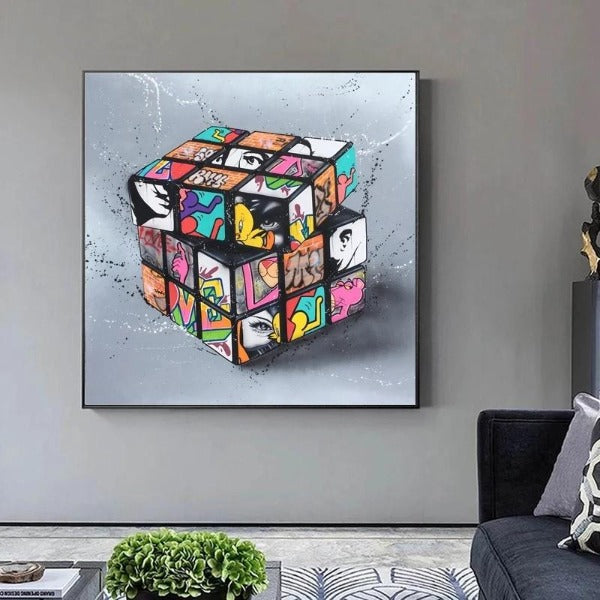In this color photograph of a living room, a prominent framed picture hangs on a dark gray wall. The picture, encased in a black frame, showcases a Rubik's Cube with a light gray background featuring white and light black dotted lines. Unlike a traditional Rubik's Cube, this one is composed of small squares adorned with various images and text. Among the images, there are multiple squares featuring parts of a woman's eye, segments of Tweety Bird, and several sections of the Pink Panther. Additionally, some squares display letters forming the word "LOVE." A distinctive arrangement of the cube shows the top row moved diagonally, with the edges and corners of each square appearing black. To the right of the picture, a black sofa is visible, adorned with gray, white, and black pillows. In front of the sofa stands a gray table with a green plant on it, complementing the gray carpet that covers the floor.